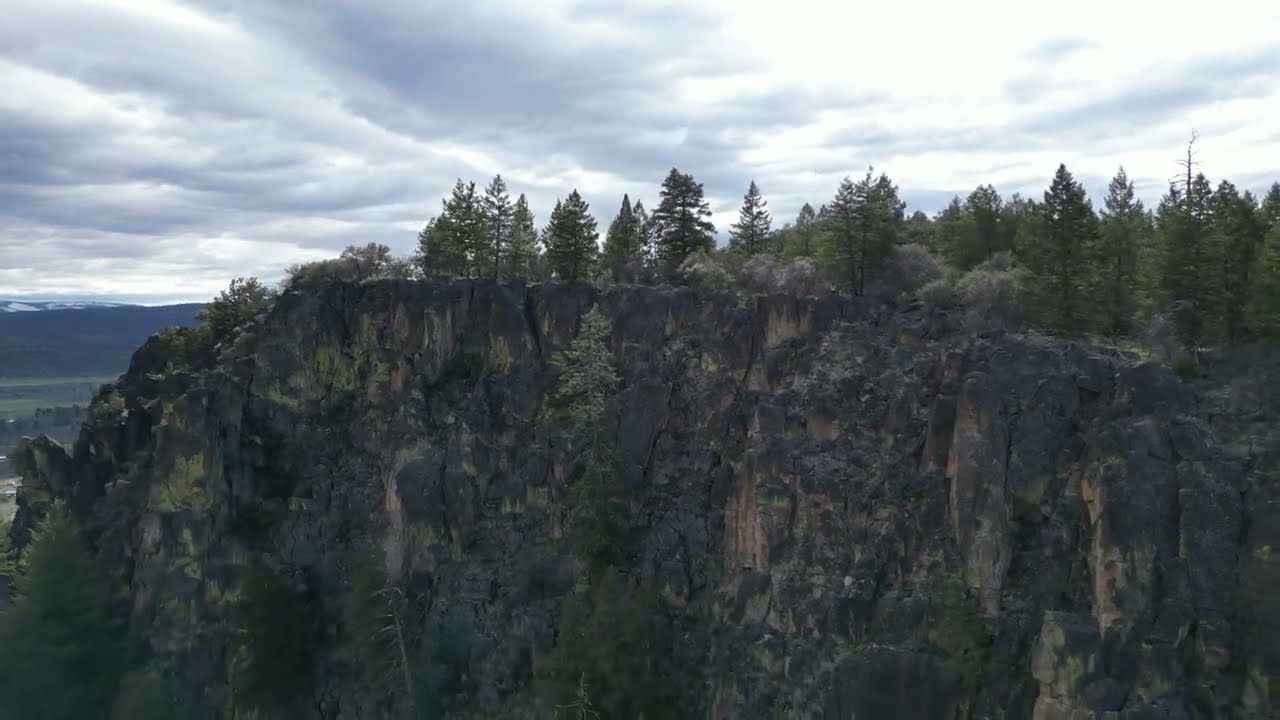The image is a detailed color photograph in landscape orientation, capturing the rugged beauty of a high cliff area. The cliff, which starts about a third of the way down the photograph and extends to the bottom, features a sheer, dark gray rock face with possible patches of moss and evidence of rock falls. At the top of the cliff, a row of vibrant evergreen pine trees stretches from the right side of the image to about three-quarters across, growing in various shades of green, from lighter hues to a vibrant, deeper green.

To the left, the cliff wall curves downward, revealing a distant view of a blue mountain range and a green grass valley, adding depth to the scene. Above, the sky is filled with stormy, dark gray, and white clouds, layered in a radial pattern, hinting at impending rain. Further in the background, additional elevations are visible, suggesting the presence of remnant hills that have eroded over time. The overall mood of the image, captured with a touch of photographic realism and representationalism, conveys the timeless, rugged beauty of natural landscapes, encapsulated in a moment of potentially changing weather.